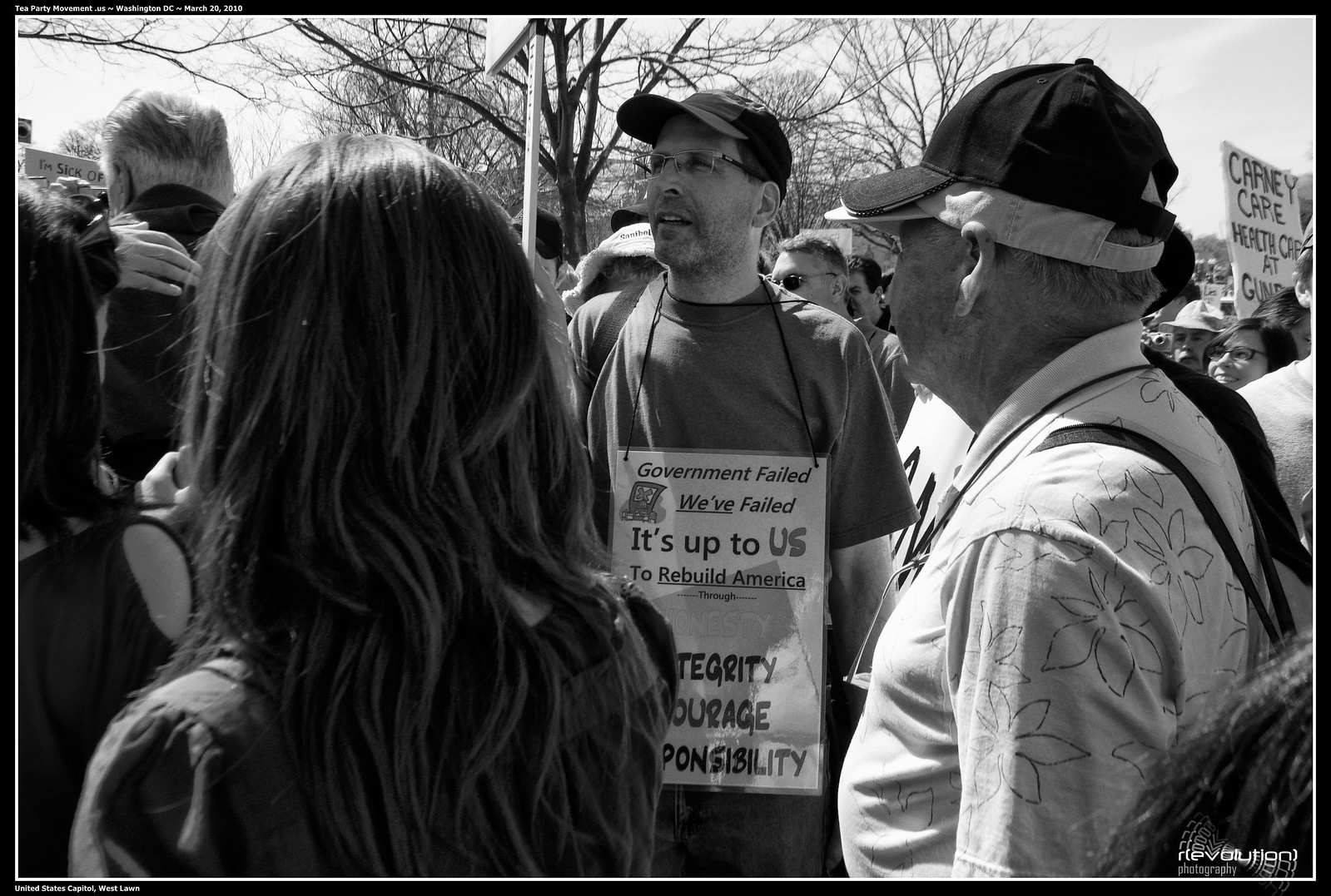In this black-and-white photograph, a diverse group of protesters stands outdoors, voicing their dissent. The central figure is a tall, middle-aged Caucasian man wearing a black cap, glasses, and a dark-colored, short-sleeved t-shirt. He prominently displays a laminated board hung around his neck, bearing the inscription: "Government failed, we have failed, you have to rebuild America." Below this text, partially obscured, are the words "integrity," "courage," and "responsibility." Flanking him are a long-haired woman on the left and a man with a backpack and cap on the right. The background reveals more protesters, hinting at a larger gathering. The photograph, emphasized by its monochrome palette, contains an icon with the word "Revolution" in the bottom corner, underscoring its message and context.